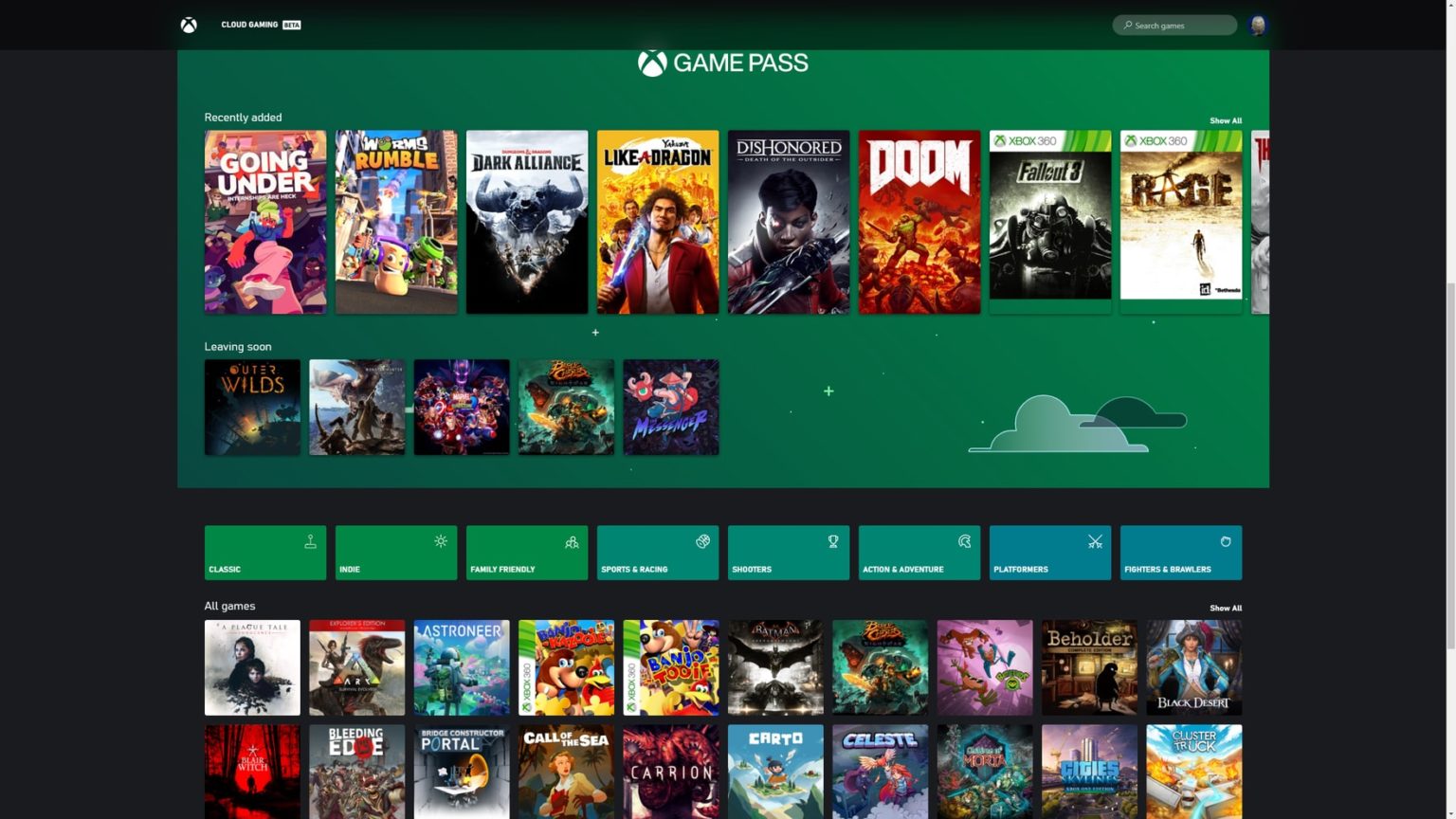This image displays the web interface for a Game Pass service, likely associated with PlayStation or Xbox. The background is black, providing a stark contrast to the vibrant, greenish-hued menu that occupies the foreground. Prominently featured are 10 to 15 video game cover images, each accompanied by the respective titles below them. Beneath this main section, there are eight small, rectangular tabs, each with text that is too diminutive to be legible. Further down, an array of smaller game cover images with their titles can be seen, offering a glimpse into the extensive library available through this service.